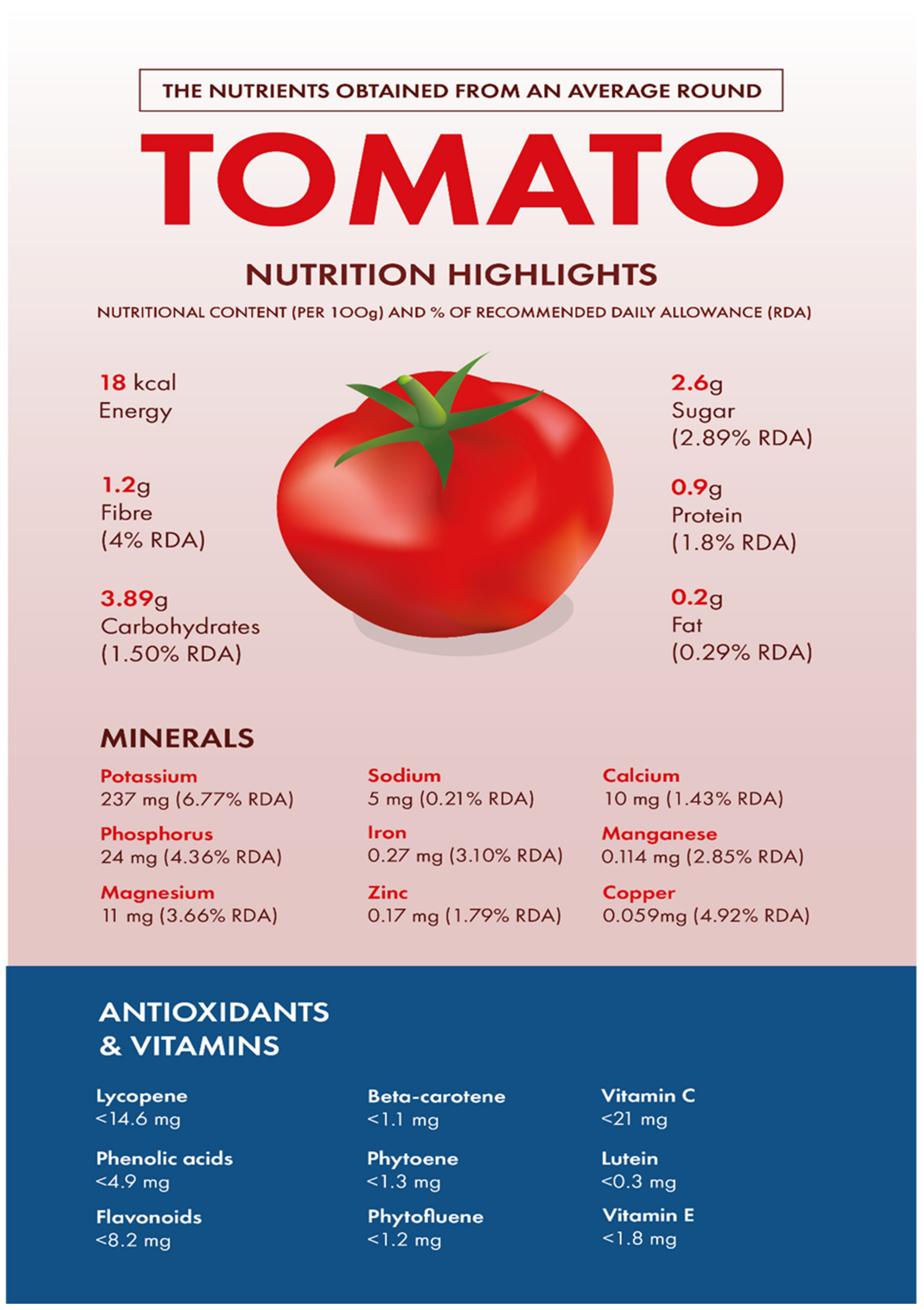The image showcases a detailed poster titled "The Nutrients Obtained from an Average Round Tomato" with the subtitle "Nutrition Highlights." Set against a light pink background, the central focus features a vibrant red tomato with green leaves. The layout is designed with the nutritional content specified per 100g alongside the percentage of the recommended daily allowance (RDA).

On the left side of the tomato, the nutritional information includes:
- 18 kcal of energy
- 1.2g of fiber (4% RDA)
- 3.89g of carbohydrates (1.50% RDA)

On the right side of the tomato, additional details provided are:
- 2.6g of sugar (2.89% RDA)
- 0.9g of protein (1.8% RDA)
- 0.2g of fat (0.29% RDA)

Further insights into the mineral content are listed below, detailing:
- Potassium: 237mg (6.77% RDA)
- Sodium: 5mg (0.21% RDA)
- Calcium, phosphorus, iron, magnesium, zinc, and copper are mentioned without specific values.

At the bottom, a section is dedicated to antioxidants and vitamins, emphasizing the comprehensive nutritional benefits of tomatoes. The title "Tomato" is prominently displayed in red text, while "Nutrition Highlights" is presented in a similar burgundy color, creating a visually cohesive and informative presentation.